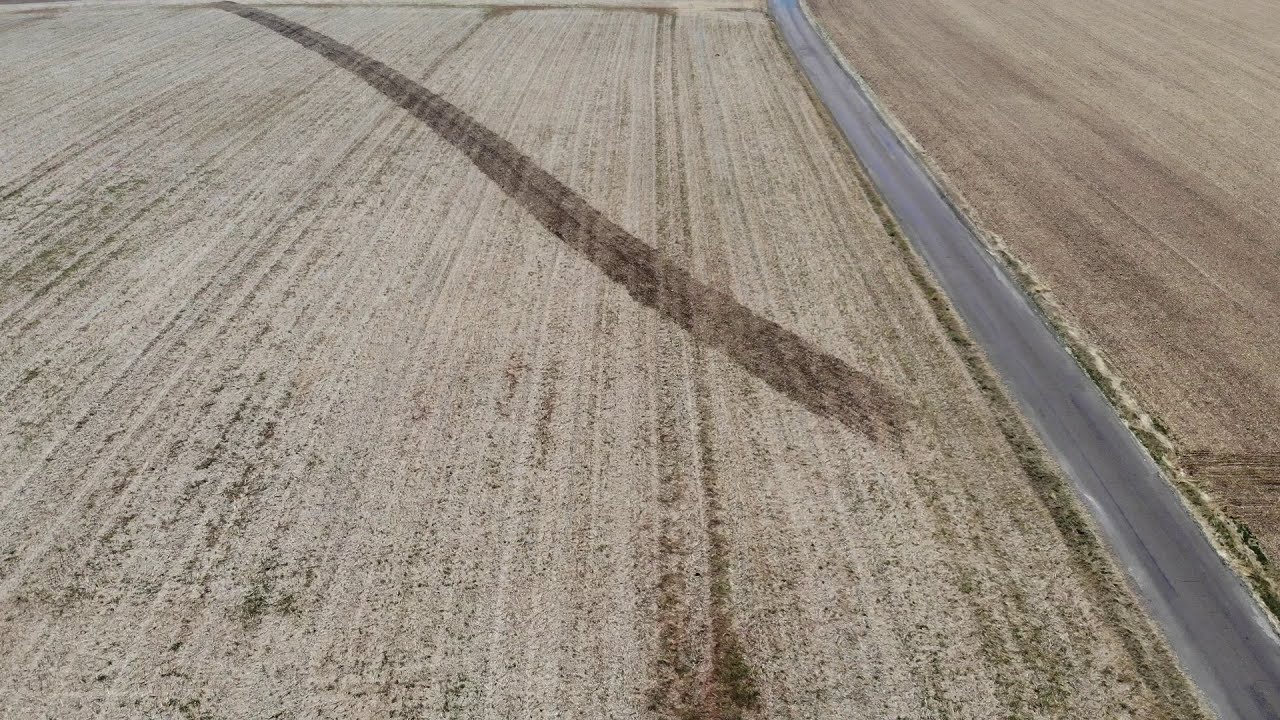The image showcases a gray, asphalt road that runs from the bottom right corner diagonally to the top center of the picture, bisecting cleared, light brown fields on either side. The road is a narrow, single-lane roadway without any markings. Both fields are distinct with vertical tilling lines indicating agricultural activity, and the field to the left of the road occupies a large portion of the image. Notably, a long, diagonal streak disrupts the neat rows in the left field, suggesting that a vehicle, likely a tractor, has driven from the lower right towards the upper left, cutting across the terrain. This dirt trail contrasts sharply with the otherwise orderly appearance of the fields. The scene is captured during daylight, highlighting the simple, nondescript yet meticulously maintained farm landscape.